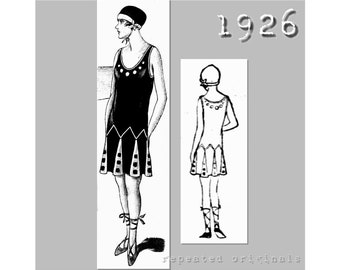This is a detailed black-and-white illustration showcasing front and back views of a 1920s flapper-inspired bathing suit. In the upper right-hand corner, '1926' is prominently displayed in white letters. The image background is gray, while the swimsuits, resembling old-fashioned dresses, are primarily black but feature distinct white elements. 

The left side of the image depicts the front view of a woman in a stylish black swimsuit that includes a black and white striped skirt falling just above her knees. The waistline of the swimsuit is accentuated with triangular shapes. She wears a black swimming cap with a white line near her forehead and shoes reminiscent of ballerina footwear that lace up her lower legs. 

On the right side, the back view of the outfit is illustrated, presenting similar detailing with a sketch-like style. The woman's hat features a strap under her chin. In both views, the swimsuit design is cohesive, combining elements like pleated skirts and geometric waist details. At the bottom right corner, there is some text which is too small to decipher, possibly indicating the source or artist of the illustration.